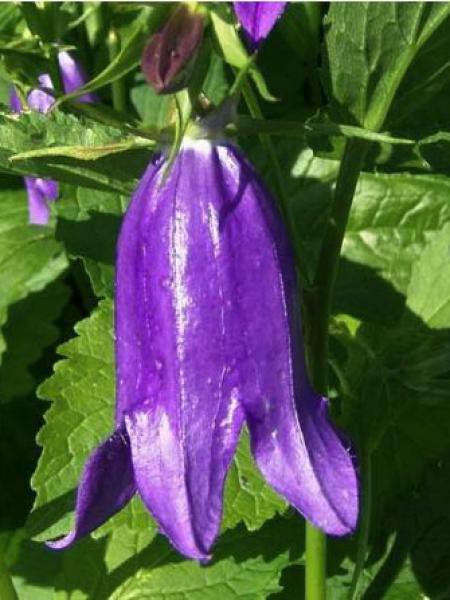In the image, the focus is on a vibrant purple flower, centrally positioned and slightly towards the bottom. The flower, resembling a bell or an upside-down eggplant, exhibits a unique shape where it splits into three distinct leaflets at the bottom. Surrounding the flower is a lush array of greenery, consisting of bright, pointy leaves that reflect sunlight, indicating a dry condition. Dark green leaves dominate the background, giving the appearance of dense brush or a garden setting. Scattered around are small unopened purple buds, adding depth and contrast to the scene. The overall color palette includes various shades of green, light purple, brown, and hints of black, creating a rich, natural tapestry. There is no visible sky or ground, ensuring that the viewer's focus remains on the intricate details of the flower and its immediate surroundings.